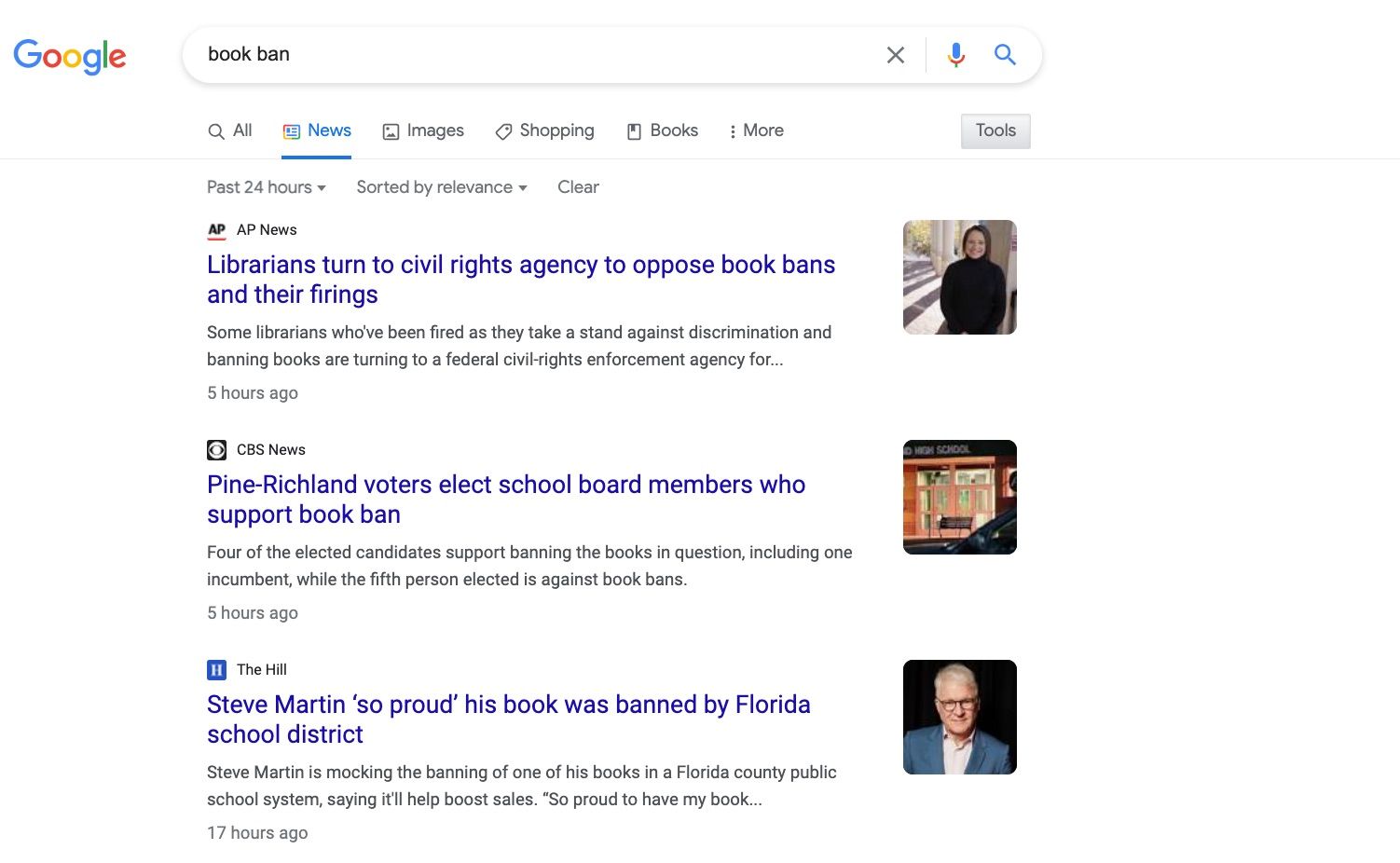This image is a screenshot of a Google search results page with a white background and no border. At the upper left-hand corner, the colorful Google logo is prominently displayed, followed by a search bar that features an X icon, a microphone icon, and a search icon. In the search bar, the phrase "book ban" is typed. Directly below the search bar is a topics menu offering various options: "All," "News," "Images," "Shopping," "Books," and "More," with a "Tools" button situated at the right-hand side. The "News" option is highlighted and underlined, indicating that it is the active tab.

The search results are presented in a vertical list, each with bold, dark blue clickable titles linked to their respective websites. The three featured search results originate from distinguished sources: AP News, CBS News, and The Hill. To the left of each article's title is a tiny snippet of text, while to the right, varying images accompany the results.

1. The first search result from AP News includes a photograph of a woman and is titled "Librarians turn to civil rights agency to oppose book bans and their firings."
2. The second result from CBS News features an image that appears to depict a library and is headlined "Pine Richland voters elect school board members who support book ban."
3. The third listed article from The Hill showcases a small portrait of Steve Martin and bears the title "Steve Martin, so proud his book was banned by Florida School District."

Each article title is clickable and designed to redirect users to the full stories on their respective news websites.